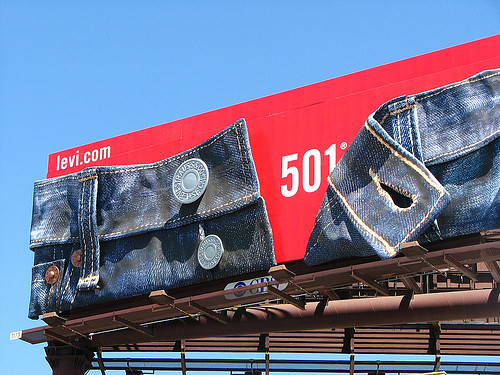This is a color photograph of an advertising billboard taken from below, set against a vibrant, cloudless blue sky. The billboard itself prominently features a vivid red background displaying "Levi.com" in the upper left corner and "501" in large white letters, accompanied by a registered trademark symbol. The standout feature of the ad is a striking depiction of a pair of Levi's 501 jeans, arranged to appear three-dimensional with the top two buttons unfastened. The left flap, complete with buttonholes, hangs down with the large, iconic brass buttons casting realistic shadows. The photorealistic denim material, detailed with gold stitching, seems to extend beyond the billboard, enhancing the impression of depth. Supporting the billboard is a rust-colored metallic structure, consisting of a platform-like scaffolding that spans from the upper right to the lower left, with visible gaps allowing glimpses of the blue sky behind. This meticulously crafted advertisement cleverly combines visual elements to create a captivating and dynamic promotion.